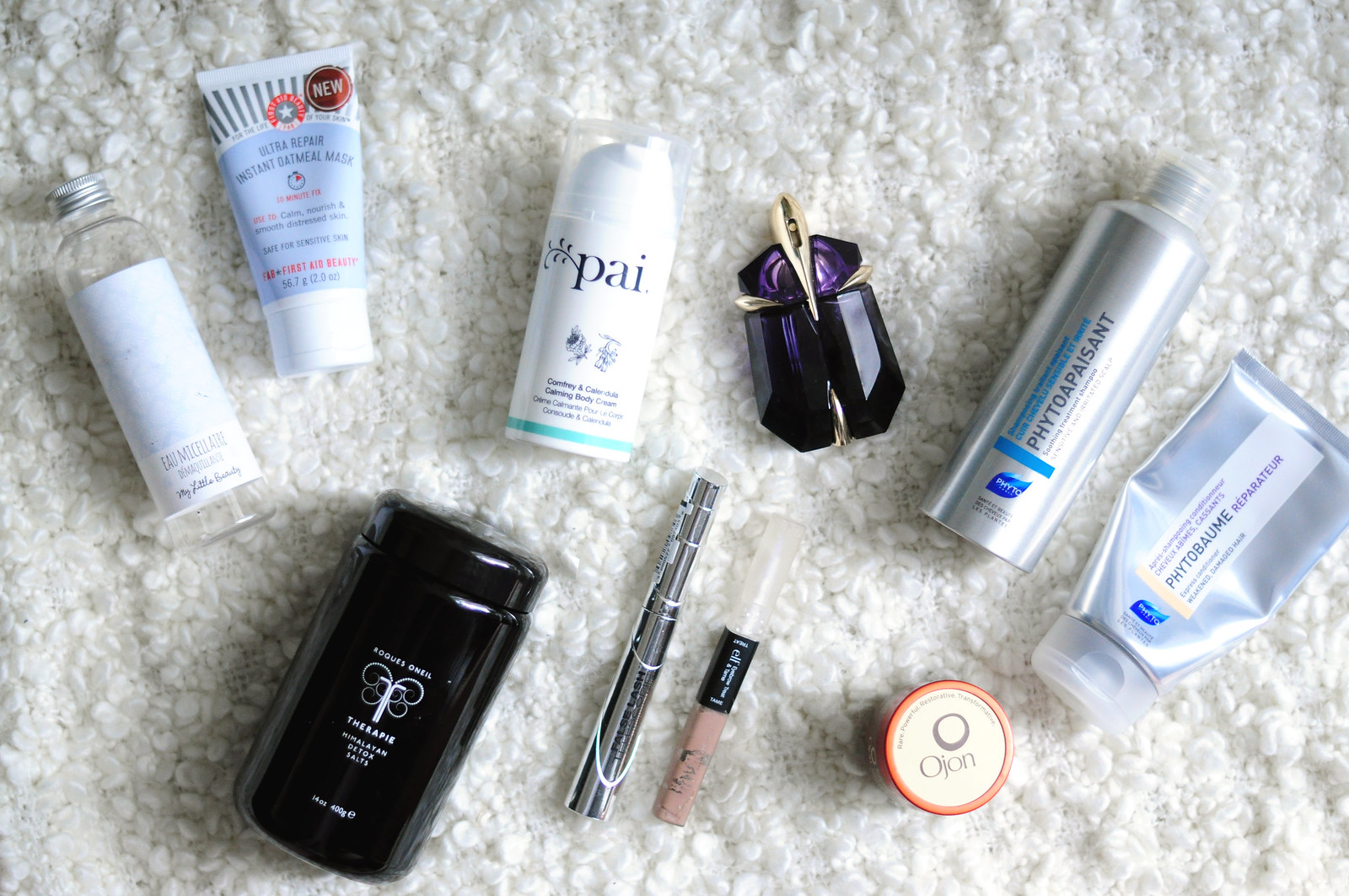The image depicts a collection of personal care items and makeup products scattered on a white rug or carpet. Among the items, there's a tube of Ultra Repair Instant Oatmeal Mask and a product labeled PAI My Body Cream. A dark purple and gold bottle, likely containing cologne or perfume, stands out prominently. Additional items include what appear to be shampoo and conditioner bottles, as well as a stick of deodorant. The assortment is completed with a tube of mascara and a lip gloss or lipstick, suggesting a mix of facial cleansing items and beauty products.